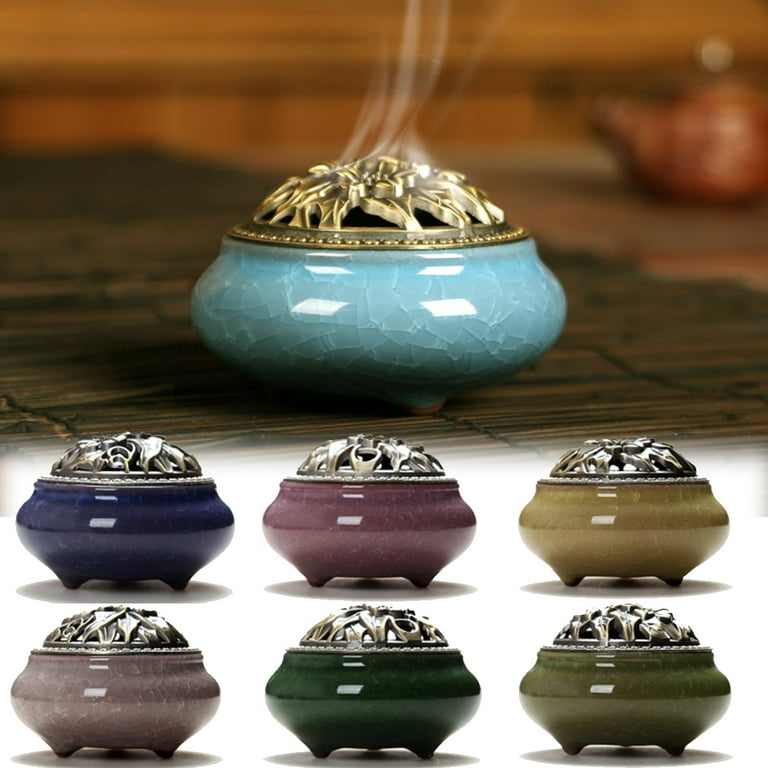The photograph showcases an artistic and detailed arrangement of ceramic incense burners. The main feature of the image is a prominent turquoise ceramic incense burner positioned at the top center. This piece, resembling finely cracked porcelain, is adorned with a rounded, circular gold metal top featuring a delicate leaf design. Wisps of white smoke emanating from it suggest it's currently in use. The burner rests atop a brown wooden stick tray, and the blurred backdrop reveals hints of a copper teapot in the upper right corner, adding a touch of rustic charm.

Beneath this focal incense burner are two perfectly aligned rows of additional burners, each exhibiting a variety of colors – deep blue, rose pink, light green, dark green, golden yellow, and beige. These burners share a similar rounded shape with metal tops designed for the ascent of aromatic smoke. The composition, with its rich details and array of colors, evokes the feel of a high-end advertisement showcasing these elegant incense diffusers in a product catalog.